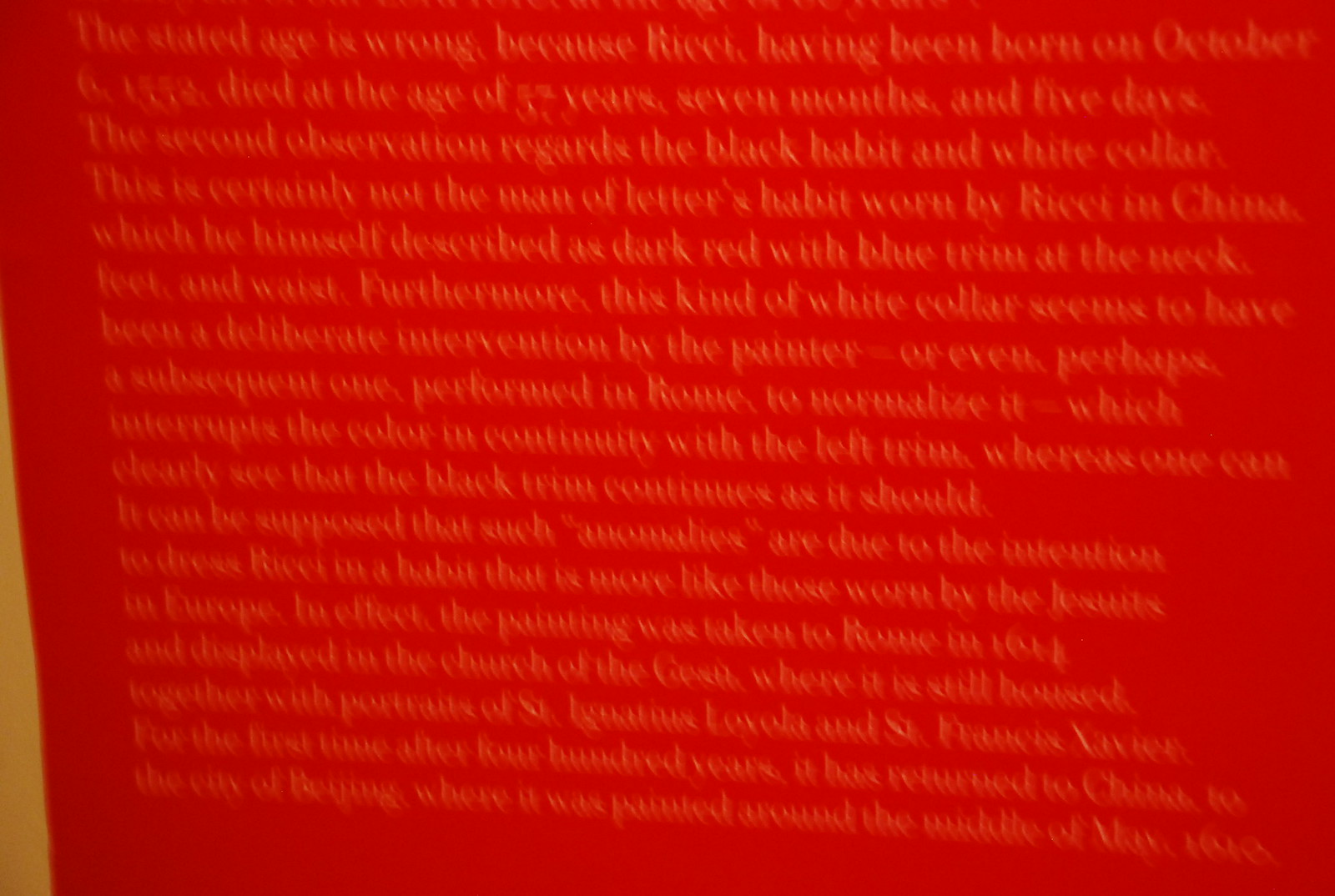This image features a predominantly red background with a subtle, artistic detail. In the bottom left corner, a strip of yellow-gold ascends from the base, only to disappear off the edge about halfway up, adding a touch of contrast and intrigue. The red area appears uniformly solid at first glance, but closer inspection reveals faint, blurred white writing. This writing is barely visible and highly unobtrusive, creating a mysterious layer of depth. The text itself is neatly aligned along a margin on the left-hand side, though the right side is jagged, with some lines extending further than others, enhancing the image’s abstract quality.